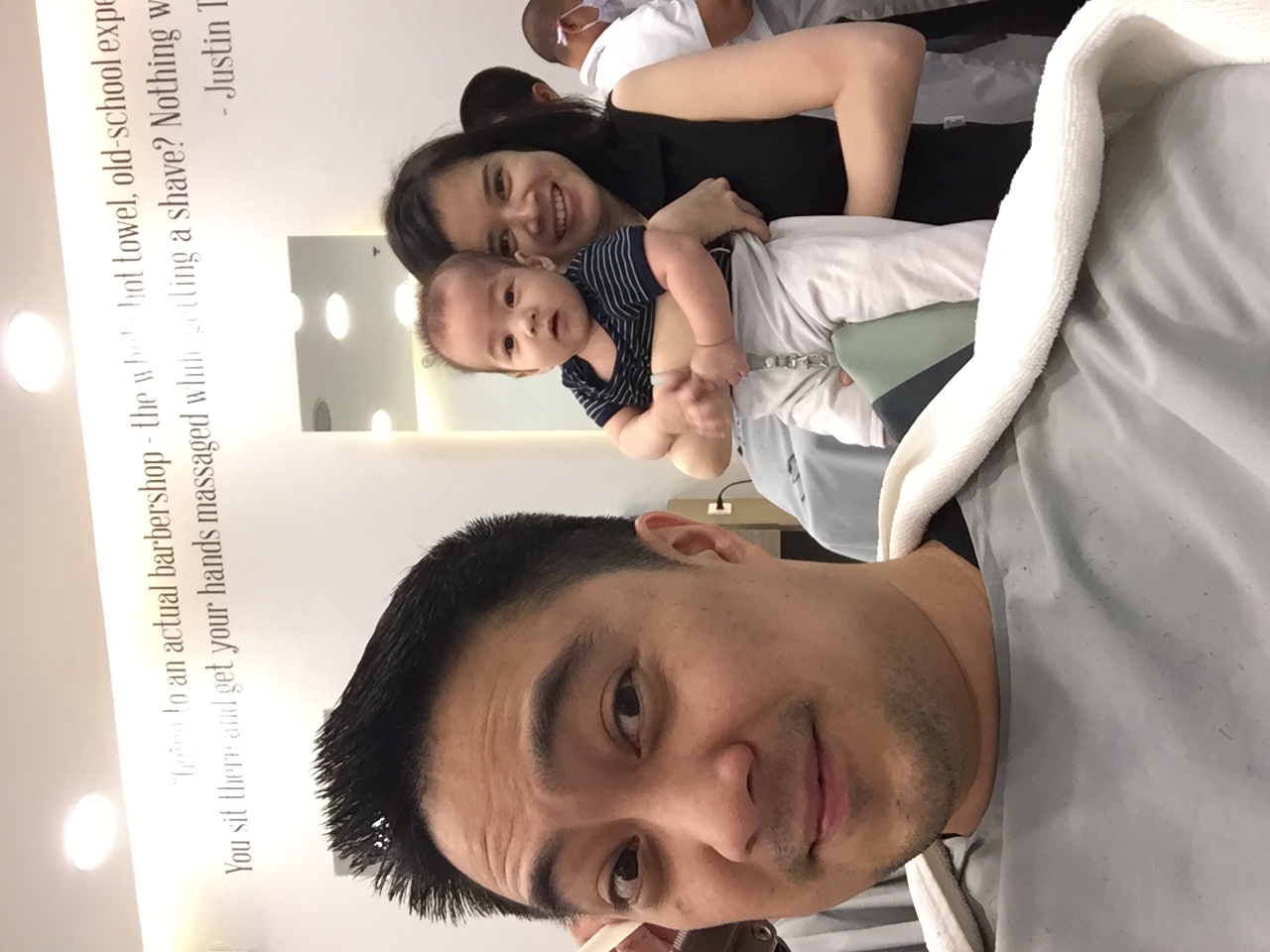In the photograph, an Asian man is capturing a selfie while seated in a barber chair, mid-haircut. A white towel drapes around his neck and shoulders, hinting at the grooming session. His closely-cropped hair and clean-shaven face dominate the frame, revealing a composed smile. Behind him, a young woman, presumably his wife, stands beaming widely in a black tank top. She cradles a small child, likely under one year old, donned in a black-and-white striped shirt and white pants. The baby gazes adorably at the camera. The backdrop features a white wall adorned with a large mirror, and partially visible black text, illuminated by overhead lights, reads: "actual barbershop, towel, old school. You sit, your hands massage, something shave," with a mention of someone named Justin, possibly Justin Timberlake. The family scene is further populated by another man in a white t-shirt, wearing a face mask, subtly blending into the background. A harmonious blend of gray, black, and white hues ties the scene together under warm barbershop lighting.